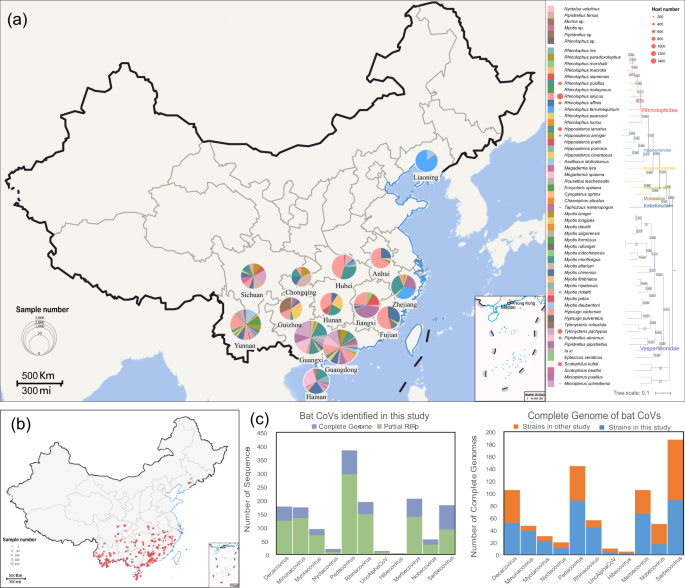This image is a detailed scientific illustration typical of what might be found in a medical or scientific journal. It comprises five frames labeled A, B, and C. Frame A, located in the top left corner, is an outline map of China, displaying all its provinces. The map includes various pie charts predominantly situated in the southeast region of China, with a key nearby explaining the significance of the pie slices, which are colored pink, yellow, red, green, and blue. These pies seem to correspond to regions and the density of certain data points.

Adjacent to this, Frame B, situated in the bottom left corner, is another outline map of China, this time featuring red dots indicating regions with a higher density of bats identified with COVID-19. 

Frame C consists of two graphs. The first graph is a line graph using green and blue lines to represent the number of bats with COVID-19 identified in the study. The axes show the provinces and the number of sequences discovered. The second graph is a bar graph depicting the number of complete genomes of bats with COVID-19, represented with blue and orange bars. Again, the x-axis lists the provinces, and the y-axis denotes the number of complete genomes.

This illustration also includes a scale converting 500 kilometers to approximately 300 miles, making it easier to gauge distances on the maps. Additionally, the image encompasses detailed yet somewhat illegible text to the right, potentially summarizing the key findings or methodologies of the study.